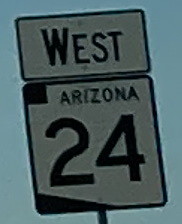This is a close-up, slightly blurry photograph of a road sign, framed almost like a postage stamp. The image is captured from a regular camera with less-than-optimal quality, and it is closely cropped, leaving little else visible beyond the sign itself. The sign consists of two parts: the top section is a small rectangular piece with curved edges, outlined in black, and features the word "WEST" in capital letters on a white background. Below this, there is a square sign that also has a black border. Inside the square, a black silhouette of the state of Arizona is prominently displayed, accompanied by the word "ARIZONA" in all capital letters above the large numerical "24." The sign is clearly mounted on a pole, visible by the screws attaching the signs to it. The background shows a dimly-lit, bluish-green sky, indicating that the photo was taken outdoors, likely on the side of a road.